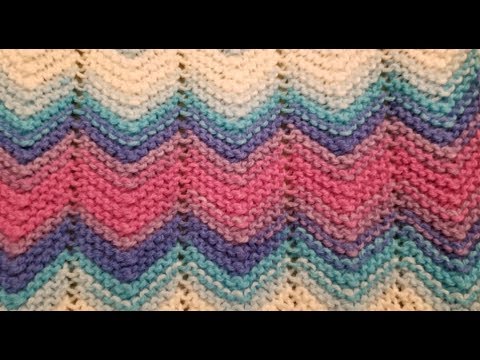This close-up photograph showcases a meticulously crafted piece of crochet, displaying a chevron pattern formed by tight, neat stitches. The design features a harmonious color palette consisting of white, pale baby blue, slightly darker blue, purple, pale pink, and bright pink, with these colors repeating in reverse order back to white. The V-shaped chevron design creates the illusion of gaps between each colorful strip. The intricate pattern and vibrant colors, which blend beautifully into one another, suggest it could be used as a decorative border on the cuffs or base of a sweater, or perhaps part of a blanket. The detailed craftsmanship and orderly stitching stand out vividly, making the fabric appear both complex and aesthetically pleasing.